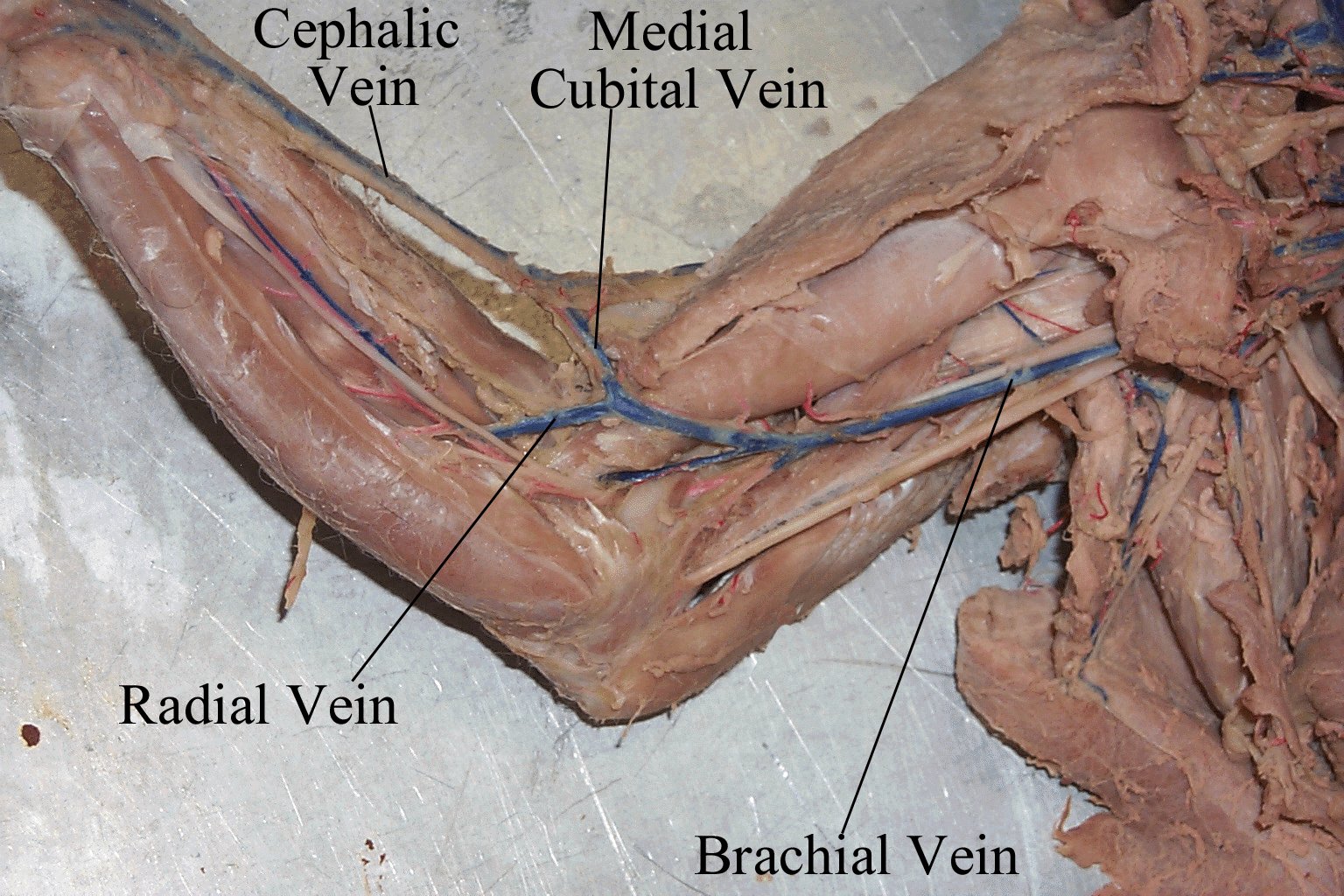The image depicts a detailed close-up of a human arm, resembling the plastinated specimens often seen in anatomical exhibits but presented in a less refined manner. The arm, with peeling and loose skin that appears an unsettling pink-gray similar to the color of raw turkey, is positioned on a rough, scratched steel surface. Distinct blue veins are visible, each clearly labeled with thin black lines connecting to their respective names: cephalic vein, which is marked in blue; medial cubital vein; radial vein as an offshoot of the medial cubital vein; and the brachial vein closer to the body. The overall appearance of the cadaver is quite disturbing and raw, exposing the internal anatomy in stark detail.